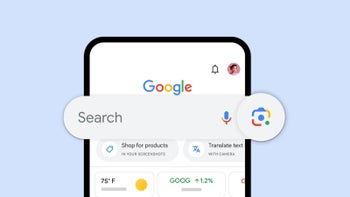The image features a light blue background on the left, right, and upper parts of the picture. Dominating the center is a phone or tablet with a black border, displaying the Google homepage. The screen showcases the iconic Google logo, rendered with two blue G's, a red E and O, a yellow O, and a green L. The notification bell and a profile picture are also visible at the top of the page.

The focus of the image zooms in on the Google search box, which takes up a significant portion of the photo. The search box itself has a grayed-out area with the word "search," flanked by a microphone icon and a camera icon for adding an image. Below the search box, there is a gray box featuring a price tag icon and the text "shop for products." To the right of this box, there is another box that is too blurry to decipher.

A horizontal line runs underneath these elements, dividing the upper search area from two white boxes below. The white box on the left indicates the current weather as "75 Fahrenheit, sunny," while the box on the right appears to show stock information for Google, noted as "GOOG +1.2%".